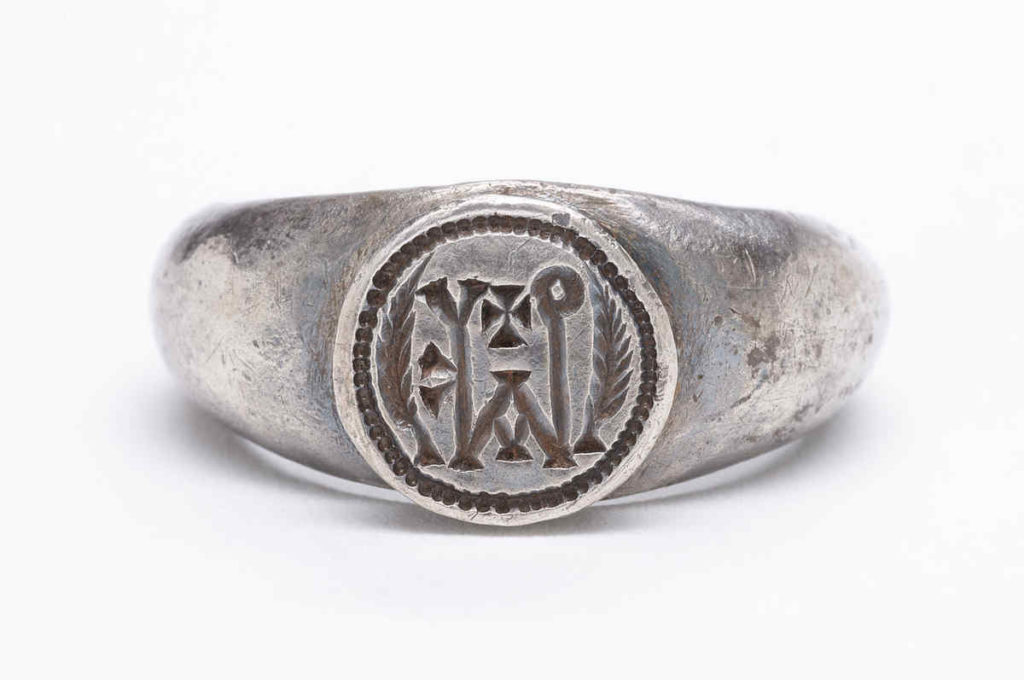The image showcases a highly detailed, antique silver ring set against a stark white background. The ring appears to be very old and carries signs of corrosion, with brown spots marring its surface. The face of the ring features a meticulously embossed circular crest. This crest is framed by an intricate rope design around its edge. Within the center of the crest, two curved leaves with individual leaflets flank a series of symbols. Prominently displayed is a black Maltese cross at its upper center. To the right of the cross is an elongated Y shape, and on the left, a vertical line topped with a circle, creating a distinctive pattern. Below these symbols, an arrangement resembling a W formed by a triangle directs upward. At the bottom, a semi-circle with what resembles bunny ears can be seen, suggesting the head of a rabbit. Despite its tarnished state, the craftsmanship of the ring reveals its age and possible historical significance, hinting at a rich, mysterious past.